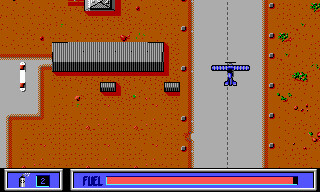This image is a screenshot of a simplistic, top-down, pixelated computer game showing a blue airplane taxiing on a tarmac. The airplane is positioned just right of center on a gray airstrip with a dotted middle line. Surrounding the runway are areas of orange dirt and sparse shrubs, giving the environment a desolate feel. There are a few smaller buildings and a much larger structure, possibly a hangar, with a notable white object in a parking lot next to it, though its details are unclear.

The interface includes a prominent blue fuel gauge at the bottom of the screen, spanning more than three-quarters of the width and indicating nearly full fuel via a red line. To the left of the fuel gauge is a small box with an icon and the number two, its function not explicitly detailed. An additional gauge or bar is present, but its purpose remains ambiguous. The visual style and environmental elements, including possible side lights and various structures, accentuate the game's rudimentary design.